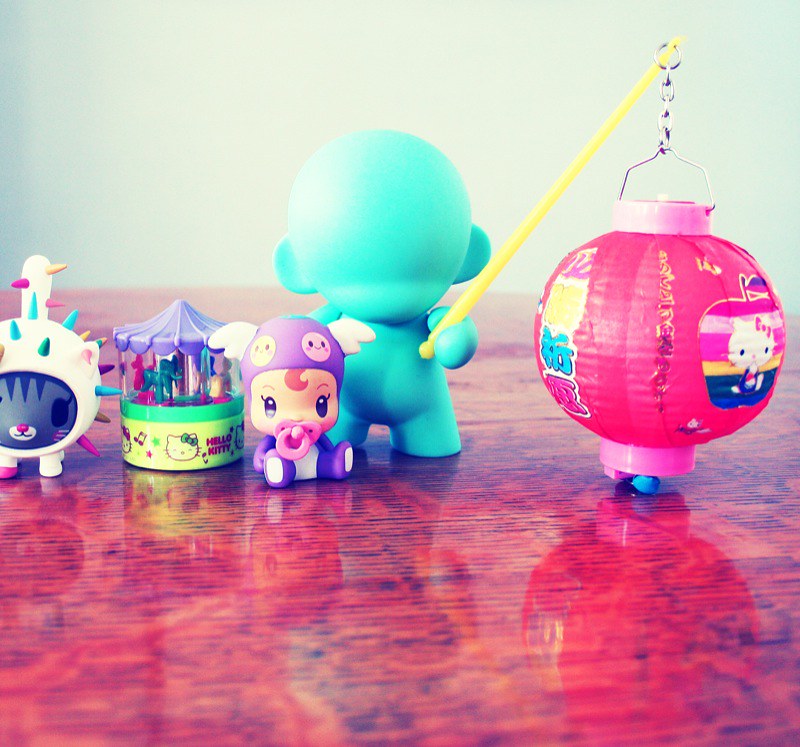This detailed photo captures a variety of children's toys meticulously arranged side-by-side on a dark wood grain tabletop, which appears red and black due to the lighting. The toys reflect off the polished surface, enhancing the scene's bright yet nearly washed-out ambiance. Against a white wall backdrop, the leftmost toy is a kawaii-style white cat with various spikes protruding from its body. Adjacent to it, there's a tiny Hello Kitty carousel. Further right, there's a small figure with a pacifier in its mouth. Another prominent figure is a blue mannequin, holding a yellow rod or stick that extends towards the upper right of the frame. This rod is attached by a chain to a large red balloon featuring the Hello Kitty logo.